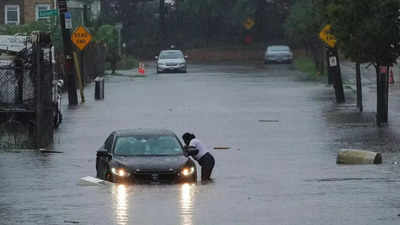The photograph depicts a completely flooded street with water covering the entire roadway. On the left-hand side, rows of houses and street light poles are visible along with a dead end street sign. On the right-hand side, there are more street poles and another dead end sign, as well as a floating barrel. In the middle of the image, a black car with its headlights on is submerged up to the headlights in floodwater. A woman, wearing a white shirt and black pants, stands bent over at the driver’s side window, possibly talking to someone inside. Her clothing and knee-deep stance in the water are clearly visible. In the background, two silver cars are parked, one on the left and one on the right, with the water not yet reaching their bumpers. The surroundings include trees, garages with old vines, and various floating objects. The image, taken either by a local experiencing the flood or a professional photographer, vividly captures the severity of the flooding, and could potentially serve as a powerful visual for news coverage.